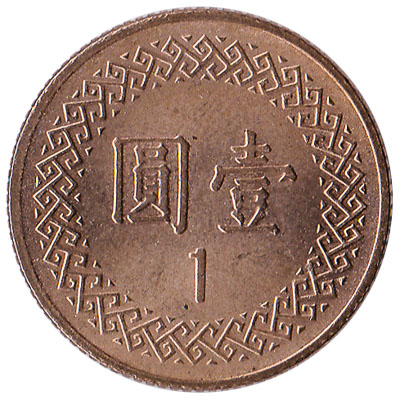The photograph showcases a bronze-colored coin viewed head-on against a white background. The coin is circular and features a slightly raised, darker brown edge with a serrated groove pattern. In the center, there are two engraved Chinese characters that spell out "Yat Yuen," a detail emphasized by all captions. Below these characters, the numeral "1" is also engraved. Surrounding the central text is an ornate, interconnected pattern of diamond shapes and lines, described variably but consistently as intricate. The surface of the coin is predominantly smooth with some darker brown hints, suggesting areas of wear or staining. This detailed ornamentation and the raised edges contribute to its intricate and visually appealing design.